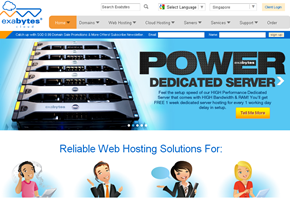This is a low-resolution screenshot of a web page laid out in a horizontal, landscape style. Despite the small size, several elements are discernable. The web page features a clean white background. In the top left-hand corner, the company name "Exabytes" is displayed, with "B-I-T-E-S" in bold. Next to the name is a logo comprising a blue cloud intersected by a wavy line that transitions from orange to blue. 

Adjacent to the logo on the right is a menu bar that includes an orange button and several grey buttons with drop-down options, though the text is too small to read. At the very top of the page, there are various input fields, including a language selection option, and a login button located at the top right-hand corner.

Below this header section is a blue horizontal banner that reads "Power Dedicated Server." Beneath this banner, some smaller blue text is visible, followed by a prominent yellow button located on the bottom right of this section. The central portion of the web page features images resembling silver server racks or other server-related hardware.

Further down, on another white background section, the text "Reliable Web Hosting Solutions for" appears in blue. This section also includes illustrative icons of various users: a boy wearing headphones and a pink shirt, a man in a business suit, a woman in a suit and tie with a blue speech bubble, and a woman with a laptop wearing a red shirt.